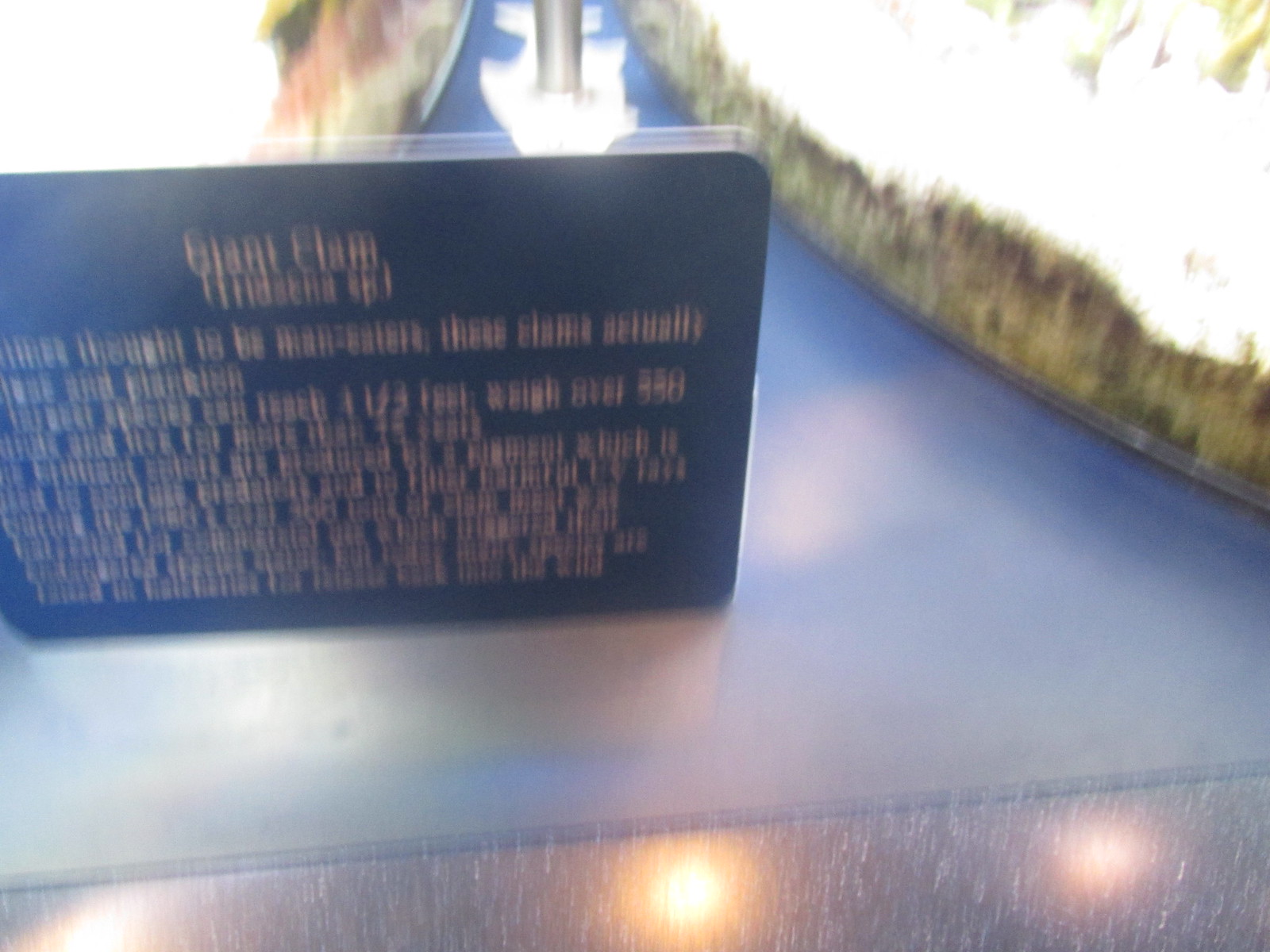The photograph depicts a blurry image of a somewhat pyramid-shaped display sign, likely situated in a museum or similar indoor space. On the left side of the image, there's a sign that reads "Giant Clam" at the top, followed by a paragraph of text detailing information about the creature, possibly mentioning its speculative reputation as a man-eater. This sign appears to be made of black marble or a similar dark material, with the text etched into the surface. The display could be part of a larger exhibit, with some kind of pole or structure rising from the base. The background includes reflections of overhead lights on a smooth, gray floor that transitions to a granite-like surface at the image's bottom. Additionally, there are hints of plant life or shrubbery on the right side, providing a mix of green, red, pink, light yellow-green, and white hues that contrast with the dark, glossy background of the sign.